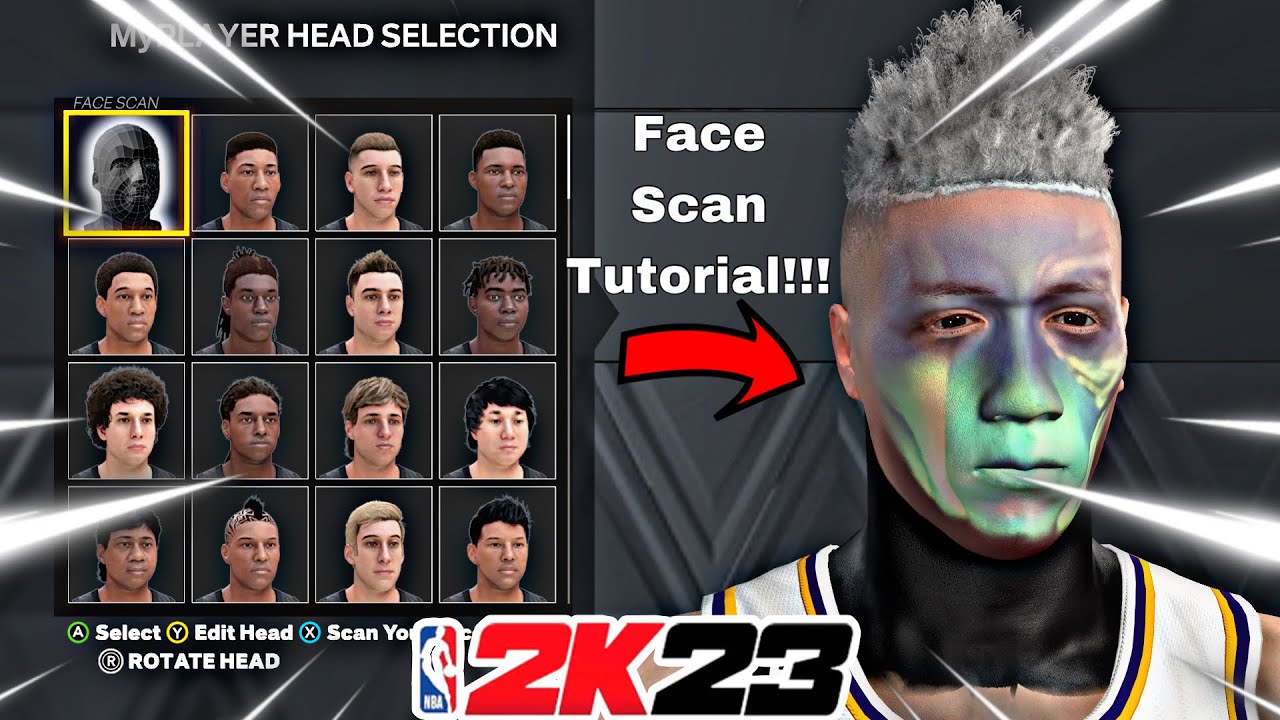The image appears to be a screenshot or web image from the NBA 2K23 video game, showcasing the "My Player Head Selection" screen. The layout is divided into two sections. On the left side, the screen is titled "My Player Head Selection," under which there are four rows, each containing four head options for customizing the player's appearance. The interface allows users to choose the facial features they want for their character.

At the bottom of the left section, several options are listed:
- Press 'A' to select
- Press 'Y' to edit head
- Press 'X' to scan your own face (suggesting the option to upload a personal face scan)
- Press 'R' to rotate the head

On the right side of the screen, there is a "Face Scan Tutorial," indicating that a user has already scanned and uploaded their face into the game. This section likely provides instructions or guidance on how to complete the face scan successfully. Additionally, there is prominent text reading "Face Scan Tutorial!!!" accompanied by a red arrow, emphasizing the feature to other players.